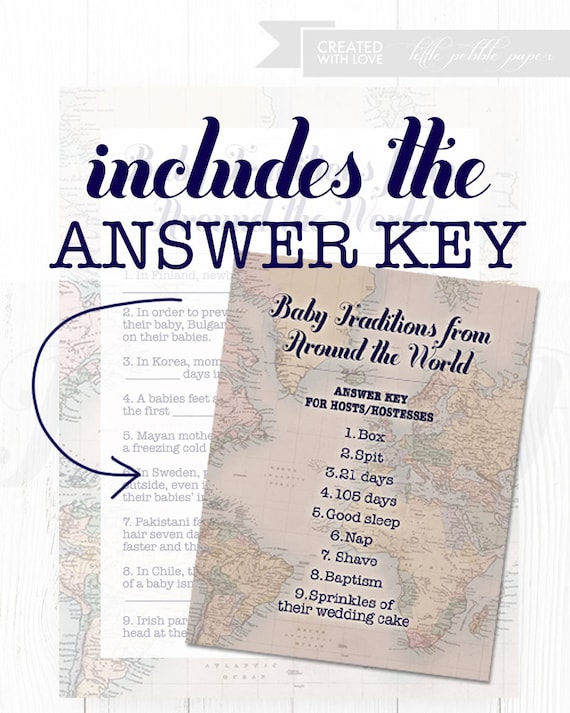The image appears to be an advertisement displaying educational materials with a theme centered around global baby traditions. In the top right corner, somewhat faint and small, is text that reads "created with love, lily, pebble, paper." Dominating the center of the image is a large blue caption stating, "includes the answer key," with a blue arrow pointing downwards. This arrow directs viewers to a prominently featured piece of paper that has the title "Baby Traditions From Around The World - Answer Key for Hosts/Hostesses."

The answer key presented on this paper includes:
1. Box
2. Spit
3. 21 days
4. 105 days
5. Good sleep
6. Naps
7. Shave
8. Baptism
9. Sprinkles of their wedding cake

Behind this main paper is another sheet with blurred text mentioning countries like Finland and Korea, possibly trivia questions related to baby traditions. Additional text snippets indicate practices such as preventing certain issues with babies in Bulgaria, and mentioning mother's days in Korea and Mayan traditions related to cold. All these papers rest on what appears to be a map, sitting on a wooden table. The background elements, including the map, are somewhat grayed out and blurry, emphasizing the clarity and prominence of the answer key and its details.